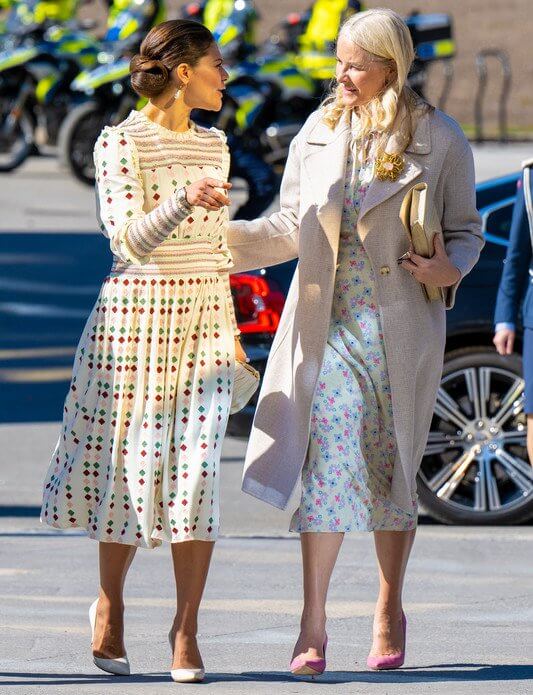This detailed color photograph, oriented in portrait mode, captures two young, well-dressed women engaged in conversation as they walk across a parking lot. The woman on the left, who has dark hair styled in a bun at the nape of her neck and wears a white dangly earring, appears to be talking animatedly, her mouth open and her right hand pointing. She is dressed in a cream-colored dress adorned with multicolored diamond patterns in red, pink, and green, complemented by horizontal striping on the top part of the dress. Her ensemble is completed with white high-heel shoes. 

To her right, the second woman, with long blonde hair, is wearing a white dress featuring colored flowers, layered under a long beige coat or trench coat. This coat is accessorized with a prominent orange brooch on the right lapel. She holds a clutch purse cupped to her body in her left hand. She also wears pink shoes. 

The background of the image includes a partially visible black car and a row of parked motorcycles, adding a sense of depth to the scene. The composition and style reflect photographic representational realism, capturing the essence of a casual, yet stylish, moment in an outdoor setting.